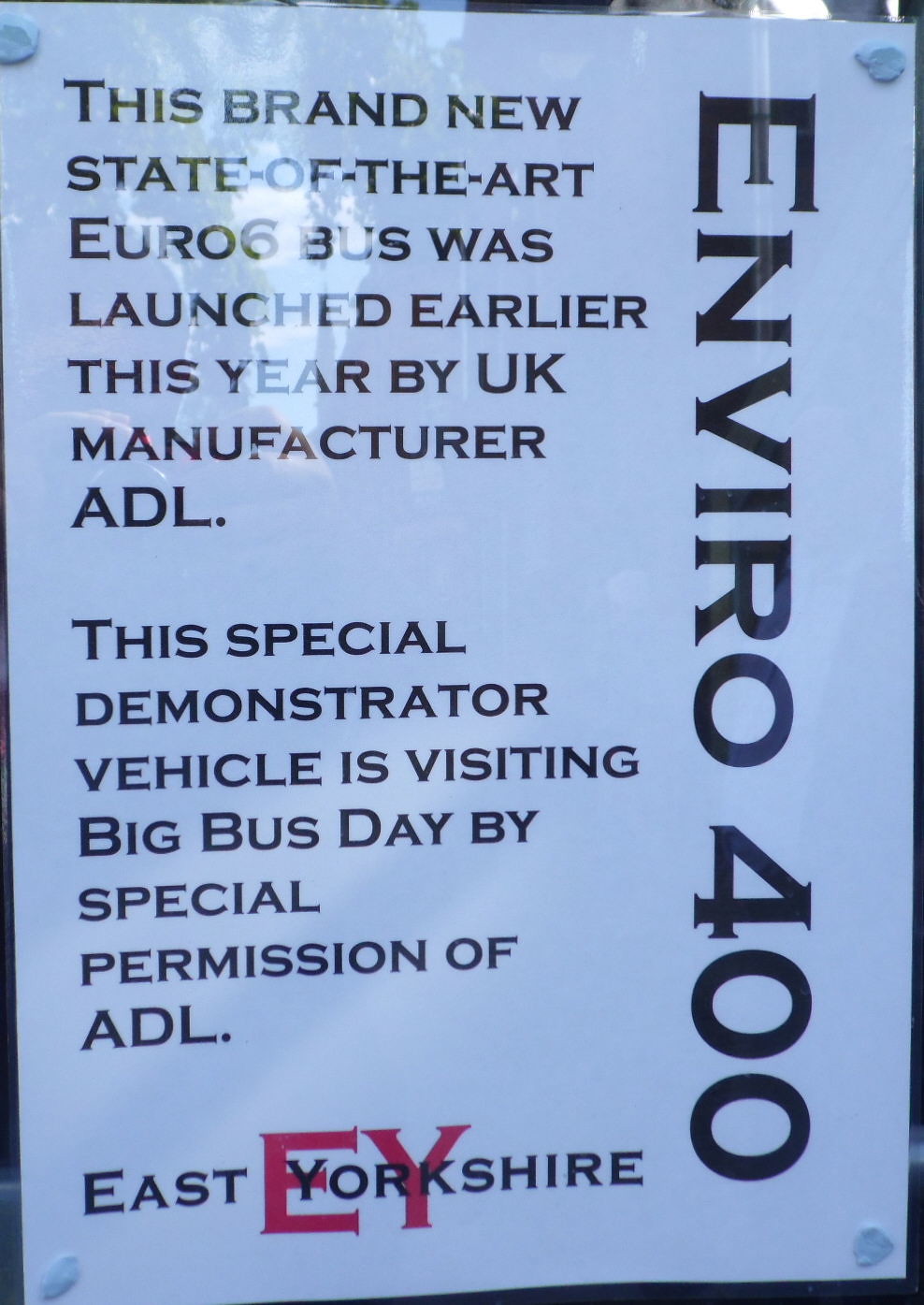This color photograph, presented in portrait orientation, features a close-up view of a white placard posted on a glass window. The placard, affixed with putty at each corner, is detailed with black text in a copperplate Gothic font. On the right side of the image, running vertically, the words "Enviro 400" are prominent. Positioned to the left of this vertical text are two paragraphs. The first paragraph reads, "This brand new state-of-the-art Euro 6 bus was launched earlier this year by UK manufacturer ADL." The second paragraph states, "This special demonstrator vehicle is visiting Big Bus Day by special permission of ADL." At the bottom left, the name "East Yorkshire" is displayed in black lettering, overlaying the initials "EY" in red. The overall style of the image is photographic representationalism realism.